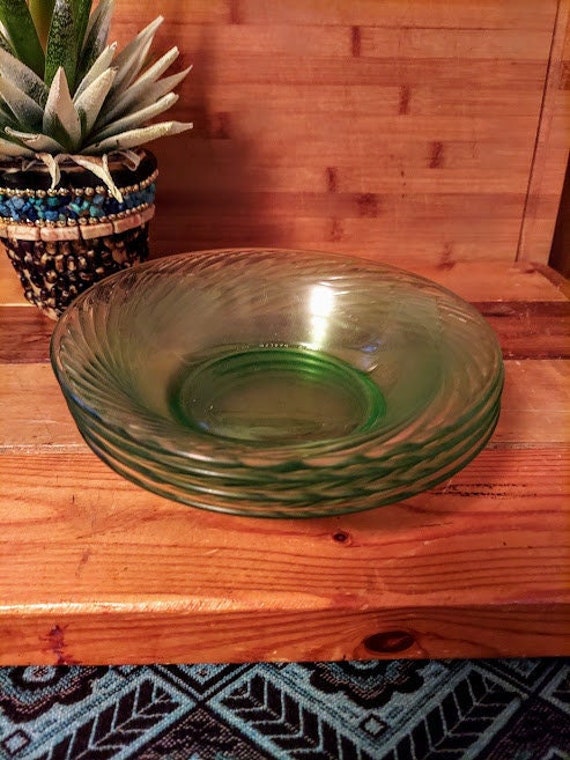A set of four identical glass dishes, each with a subtle green tint and elegant swirling lines that curve symmetrically to the right, are stacked on a light brown wooden platform. The wooden surface is approximately two inches thick and rests atop a piece of fabric adorned with gray and light blue floral patches and angular designs. In the background, a potted plant with a black base and yellow rocks sits in the left corner. The pot features a ring near the top decorated with turquoise rocks and a silver beaded line above and below the ring. The plant itself is a small cactus with both green and white leaves. The entire scene is set against a light brown wooden wall, suggesting the dishes and plant are on a shelf or mantle, possibly with decorative black and blue tiles in front.